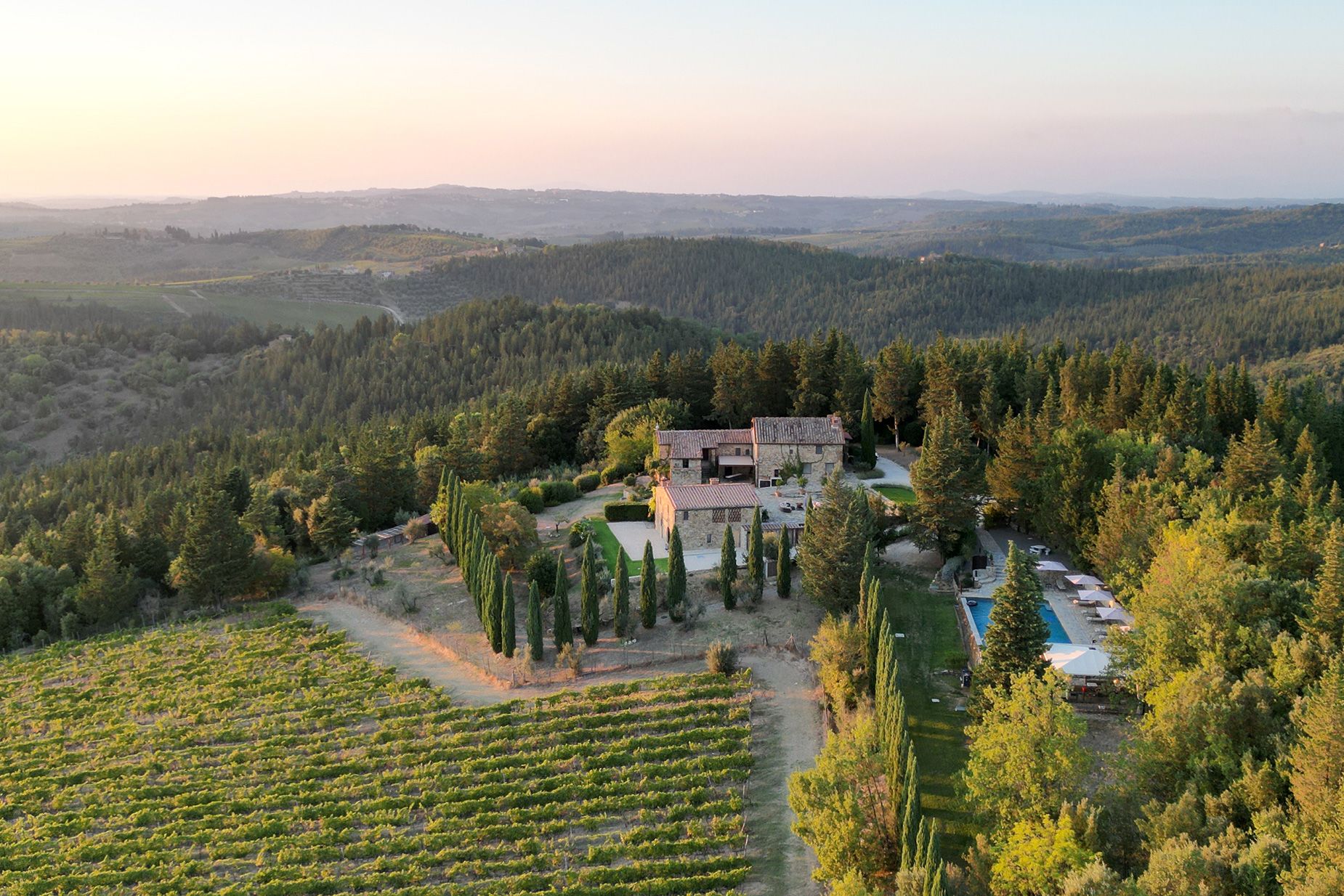This aerial photograph, likely taken by a drone, captures a sprawling mansion complex set in a scenic, outdoor setting. The central feature is a group of three interconnected white buildings with gabled, red roofs, all nestled on a concrete platform. Surrounding the mansion is a meticulously maintained landscape, including a terraced grassy slope in the foreground and a rectangular blue swimming pool, complete with several lounge chairs, positioned to the right of the houses. Encircling this property is a perimeter of lush trees, providing a natural boundary. The backdrop features majestic mountains and a forested area, adding to the sense of seclusion and serenity. The sky above is a stunning blend of blue and shades of red or orange, contributing to the overall picturesque and tranquil atmosphere. The absence of additional buildings in the distance suggests that the property is likely situated in a rural or countryside location.